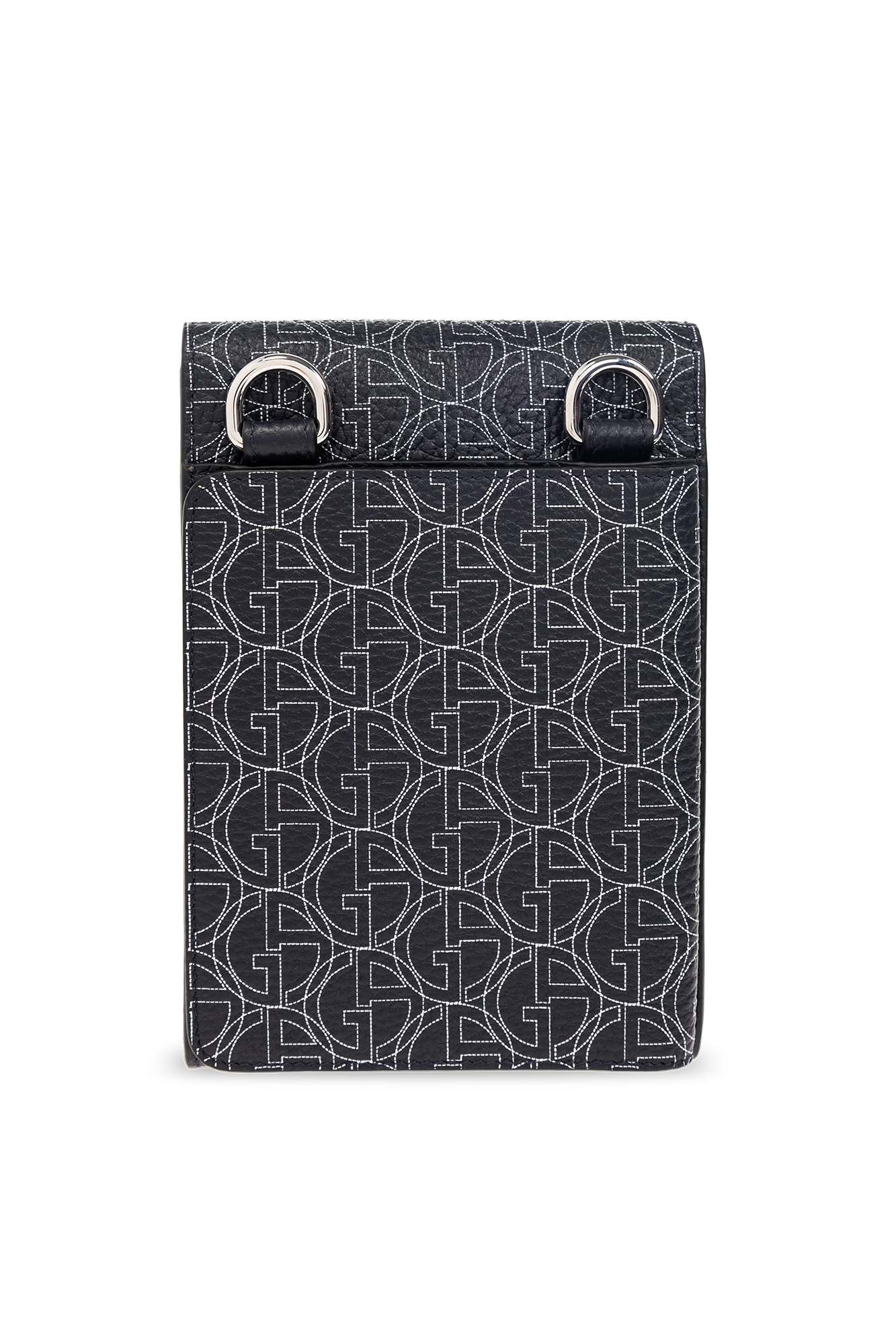This image depicts a small, black fabric pouch prominently featuring a sophisticated design. The pouch's striking black color is accentuated by a white stitched pattern that forms the interlocking initials G and A, emblematic of Giorgio Armani. These initials create a cohesive, circular design that repeats across the surface. The pouch, shaped somewhat like a business card turned upright, includes a visible pocket or opening at the top. Additionally, two silver metal buckles are attached with leather accents on either side, suggesting the presence of handles or a strap, indicative of its designer nature. The detailed photo captures the nuances of the pouch's texture and the sheen of the metal buckles.